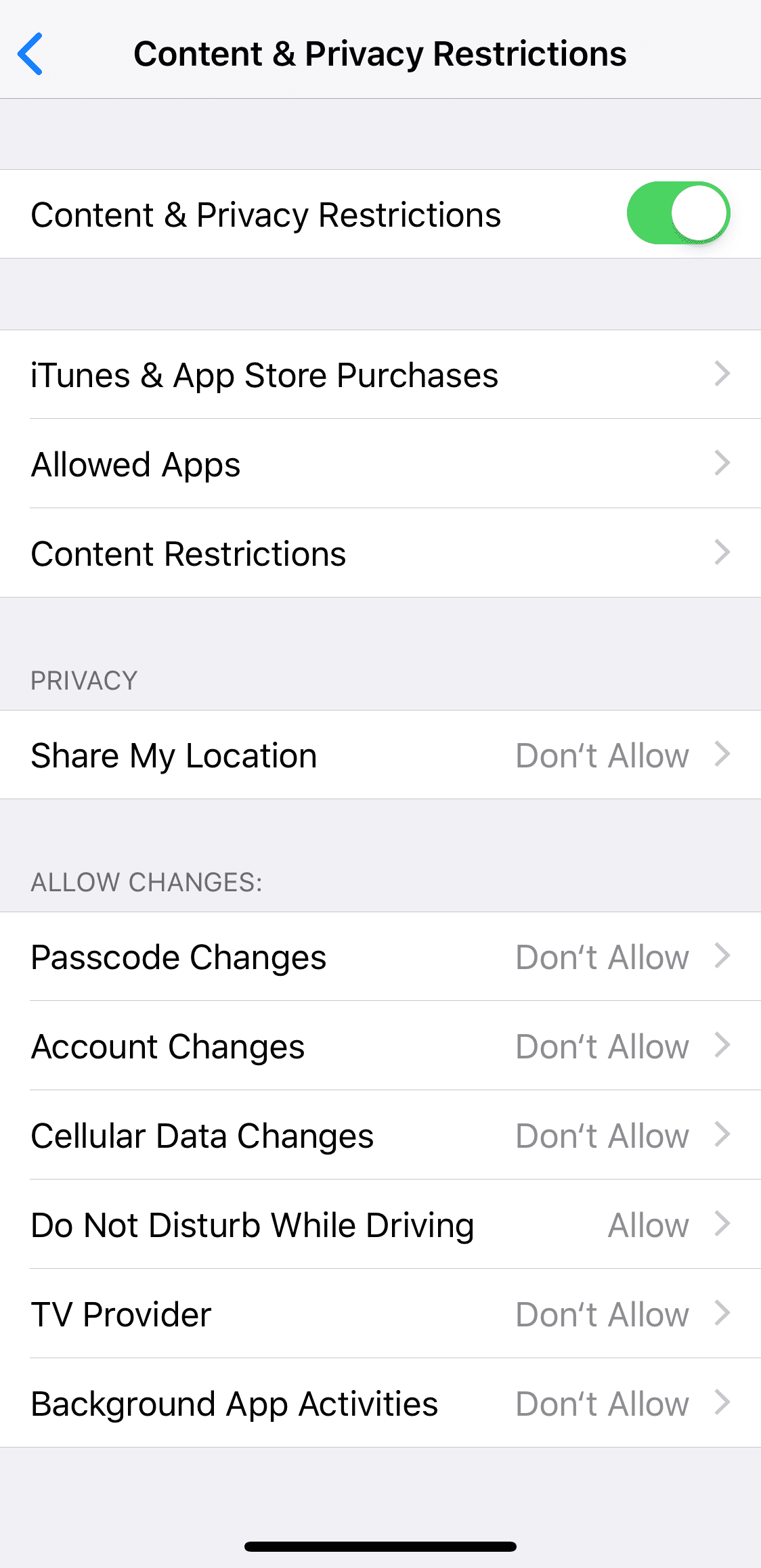This image is a screenshot taken from an iPhone, displaying the "Content & Privacy Restrictions" settings. At the very top, the heading "Content & Privacy Restrictions" is prominently shown, indicating that this feature is turned on. Below this, the menu is divided into several sections with various options, each accompanied by a gray arrow pointing to the right.

The first section includes:
- **iTunes & App Store Purchases**
- **Allowed Apps**
- **Content Restrictions**

Each of these options has a gray arrow suggesting there are further details available to explore.

The second section is titled **Privacy** and features the setting:
- **Share My Location:** Set to "Don't Allow," also with a gray arrow to the right.

The final section is labeled **Allow Changes** and lists several restrictions:
- **Passcode Changes:** Set to "Don't Allow"
- **Account Changes:** Set to "Don't Allow"
- **Cellular Data Changes:** Set to "Don't Allow"
- **Do Not Disturb While Driving:** Set to "Allow"
- **TV Provider:** Set to "Don't Allow"
- **Background App Activities:** Set to "Don't Allow"

Similar to the previous sections, all these settings have a gray arrow to the right, indicating more details can be accessed by selecting them. This organized view provides a comprehensive snapshot of the user's content and privacy preferences on the device.